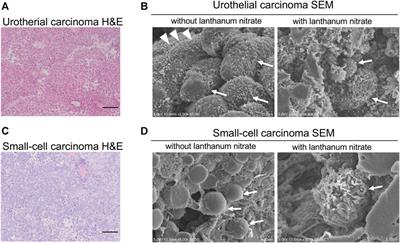The image displays a detailed scientific comparison of urothelial and small cell carcinomas using both traditional microscopy and scanning electron microscopy (SEM). The diagram is divided into four labeled sections: A, B, C, and D. 

- **Section A** (Top Left): Shows a pink-stained histological slide of urothelial carcinoma using Hematoxylin and Eosin (H&E) stain, with a small black scale bar for reference.
- **Section B** (Top Right): Contains two SEM images of urothelial carcinoma. The left image is labeled "without lanthanum nitrate" and the right, "with lanthanum nitrate". Both black and white images have arrows pointing to key features of the cells, appearing mostly gray.
- **Section C** (Bottom Left): Displays a lavender-stained histological slide of small cell carcinoma using H&E stain, also featuring a small black scale bar.
- **Section D** (Bottom Right): Features two SEM images of small cell carcinoma. Similar to section B, the left image is labeled "without lanthanum nitrate" and the right, "with lanthanum nitrate", with white arrows indicating important details in the grayscale images.

Each image provides microscopic insight into the cellular structure of these carcinomas, comparing traditional staining techniques with advanced electron microscopy.